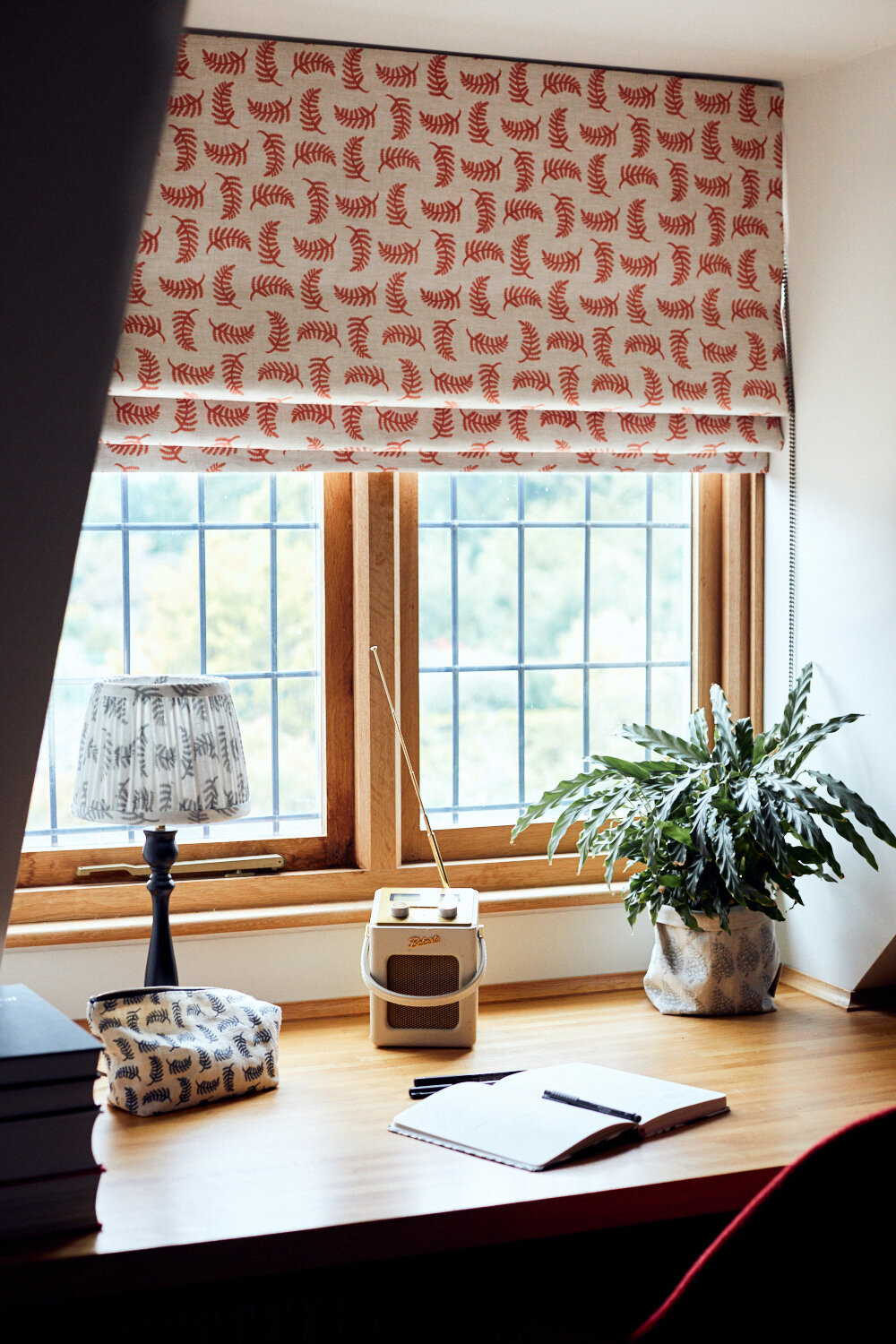The image depicts a cozy, rustic study nook within a country home. A small brown desk, nestled against large windows with natural stained wooden panes and an external metal fence, forms the centerpiece of the scene. The windows offer a serene view of a lush, forested area outside. A white curtain with a repeating red fern leaf design is partially drawn above the windows. 

On the desk, a variety of items are meticulously arranged: a little potted plant with long, green, zigzag-patterned leaves sits to the right, while a vintage white radio with a handle and antenna occupies the center. To the left, there's a thin desk lamp with a black base adorned with a white floral print, mirroring the fern motif on a nearby zippered bag. An open notebook, likely a journal, is laid out on the desk, accompanied by several pens and four thick books with black covers. The well-lit photograph, capturing the inviting and well-organized space, exudes a quaint country charm.